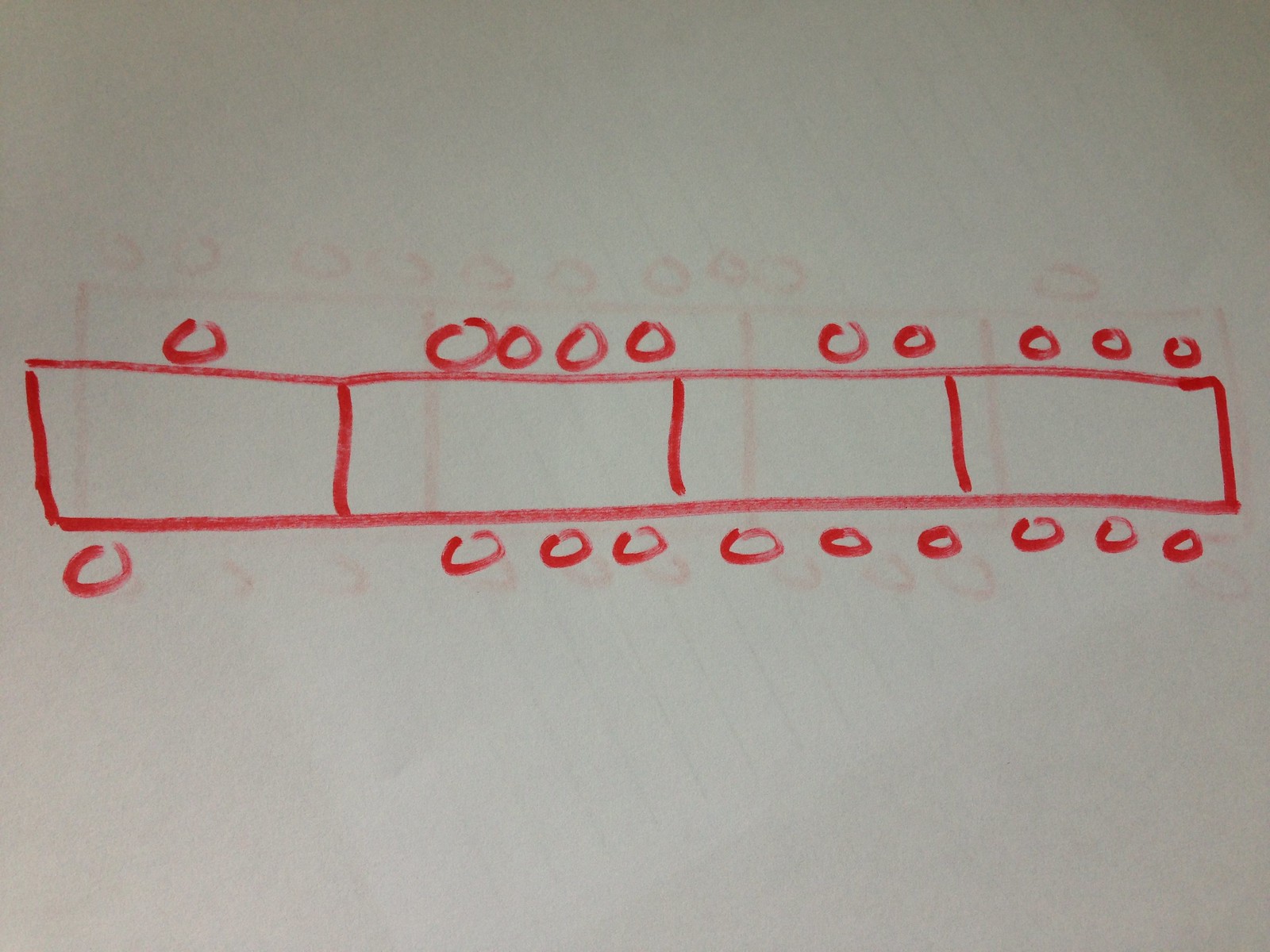This is an image drawn on a white piece of paper. On the reverse side, there's a similar image drawn in red marker that shows through, suggesting that the paper is thin. The primary drawing on this side, also done in red marker, features four sequentially connected, crudely drawn rectangles resembling boxcars of a train or parts of a segmented truck. The red marker used for the drawing appears to be drying out, as evidenced by the uneven, faded strokes visible at various points, particularly around some of the lines and circles.

Each rectangle or box is topped with circles: the first box has one circle, the second has four, the third has two, and the fourth has three. Below the boxes, there are sets of circles that could be interpreted as wheels or some form of structural detail. Specifically, the pattern beneath the boxes is as follows: under the first box, there are three circles, under the second, one circle, followed by groups of three circles under both the third and fourth boxes.

Despite the lack of neatness or precision in the drawing—it is haphazard with uneven, unaligned boxes—it conveys a sense of motion or connection, perhaps indicative of a train or a vehicle with multiple compartments. The abstract nature of the image leaves its exact purpose or representation open to interpretation, wandering between an intercom, train, truck, or some other conveyance. There are no textual labels or annotations to clarify the subject of the drawing.